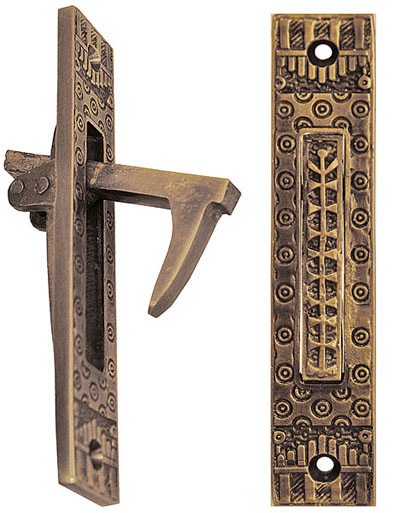This photograph features an intriguing brass object presented from two angles against a white background. The object, believed to be a vintage or antique door knocker, showcases intricate craftsmanship. The left portion of the image displays a side view, where the knocker protrudes outward, resembling a boot with a long, pointy toe aimed downwards. This portion highlights the knocker's hinge mechanism, allowing it to extend outward. Surrounding the knocker are detailed squiggly and spiral designs, adding to the object's texture and ornate appearance.

The right portion offers a head-on perspective, presenting the object in a closed position. It features a long rectangular brass plate with two holes at the top and bottom, akin to those found on a light switch cover but narrower. The surface is adorned with concentric circles and raised decorative elements, including donut-shaped engravings within the central rectangular section. The brass material exhibits shades of bronze and a Nebraska golden hue, emphasizing its vintage and possibly ancient quality. This detailed portrayal provides insight into both the functional and aesthetic aspects of the brass door knocker.